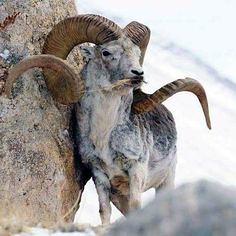The photo depicts a Big Horn Sheep standing against a rock wall on a high precipice. The animal's massive, brown horns curl back around themselves, nearly covering its entire skull and resembling double spirals adorned with black horizontal lines. The sheep's thick coat, suited for cold weather, is a mix of light and dark gray with white on its chest and is possibly shedding slightly. The Big Horn Sheep, rather small and slightly chubby, faces the camera at a 45-degree angle with its right eye looking directly ahead, chewing on a piece of grass or plant. The gray and brownish rocky wall behind the sheep adds texture, while the out-of-focus background hints at a steep, light-colored hillside. Additionally, the bottom right corner of the image is obscured by an indistinct object, masking the sheep's feet.